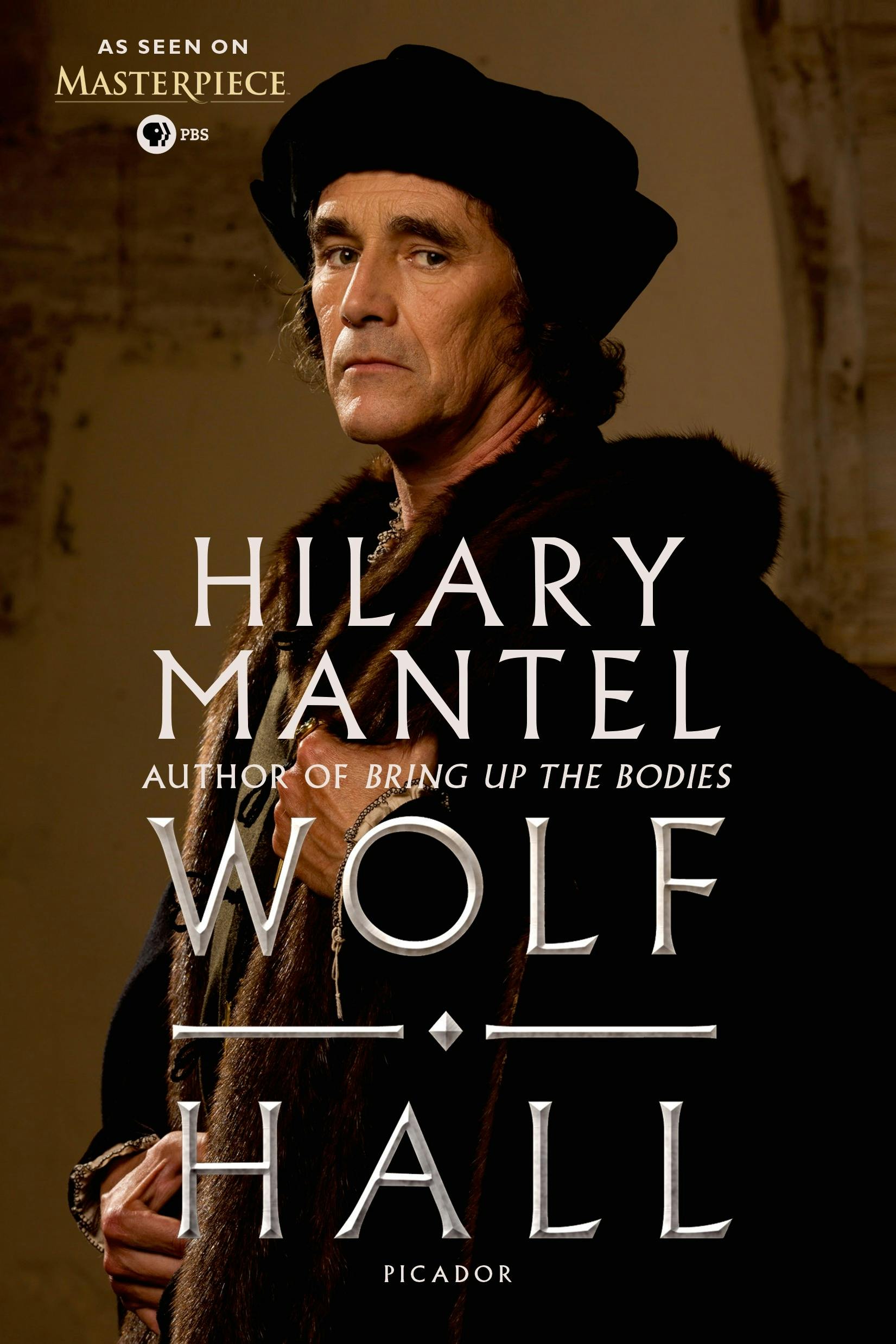The book cover for "Wolf Hall" features a striking image of a man standing against a textured old castle wall. He is garbed in a large fur coat with a black, large beret atop his head, exuding a serious demeanor as he gazes towards the viewer. His left hand is clutching the bottom of the collar of his coat, while his right hand rests across his midsection. The background has a rustic, perhaps unfinished look, with elements that seem to be made of brick, stone, or wood. 

At the top left corner of the cover, in white text, it reads "As Seen on Masterpiece" accompanied by the PBS logo, which consists of a white head overlapping a black head within a white circle. Below this, the main text overlay declares "Hilary Mantel" in prominent white letters, followed by "author of Bring Up the Bodies." The title "Wolf Hall" appears in large white text with a decorative line and diamond separating the words. At the bottom of the cover, "Picador" is printed in small white letters.

Overall, the cover blends both historical and regal elements, reflecting the thematic essence of Hilary Mantel's work.